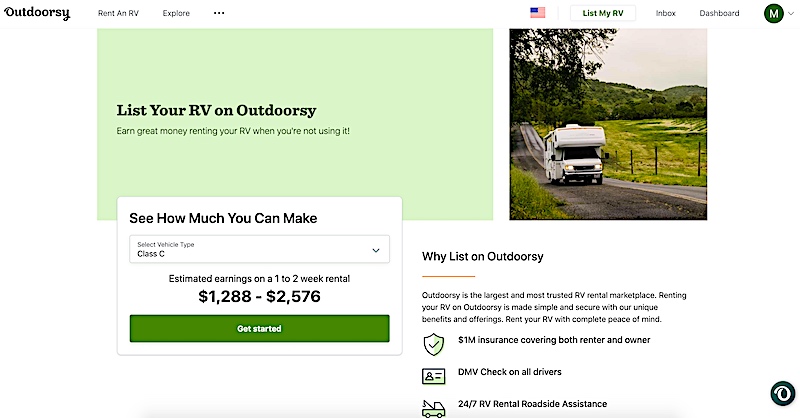The image depicts the homepage of the Outdoorsy website. In the top left corner, the Outdoorsy logo is prominently displayed. Centrally positioned is a headline encouraging RV owners to "List your RV on Outdoorsy." Directly beneath this main message, a subheading invites users to "Earn great money renting your RV when you're not using it." Below this, a secondary section features a bold call to action, "See how much you can make," alongside a dropdown menu labeled "Select vehicle type," currently showing "Class C." An estimated earnings range for a 1-2 week rental is provided, indicating potential earnings between $1,288 and $2,576. At the bottom of the section, a large, green button invites users to "Get Started."